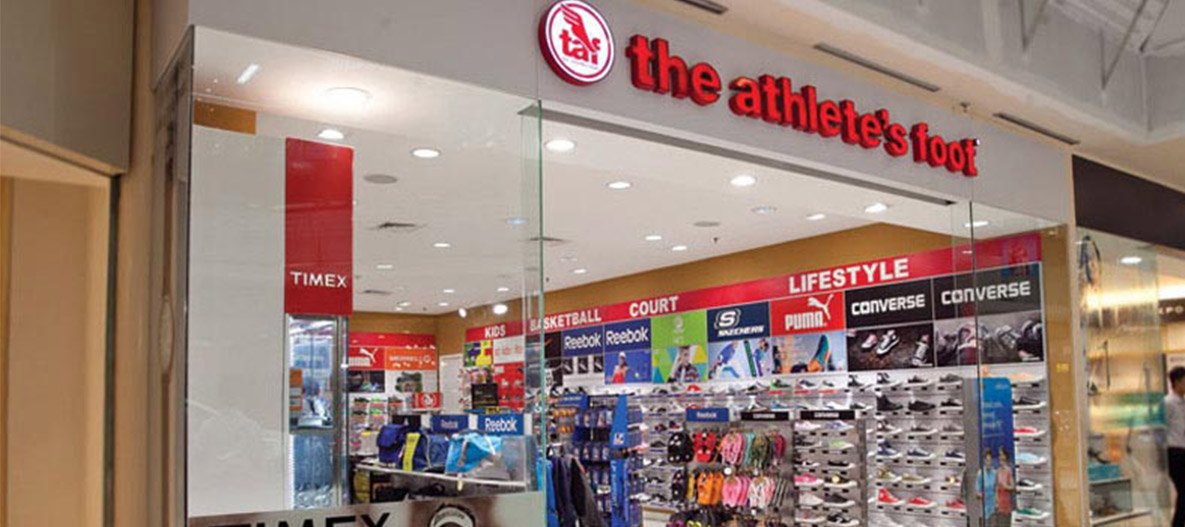This landscape-oriented photograph captures the storefront of "The Athlete's Foot" located in a mall. The store's name is prominently displayed in red letters on a gray border, situated at the top of the entrance. Adjacent to the store's name on the left side is a white circle outlined in red, featuring the letters "TAF" and a wing design emerging from the ‘F’. The storefront is composed of large glass windows and an open door, providing a clear view of the interior.

Inside, the right side of the store prominently features a red banner that lists categories such as "Kids," "Basketball," "Court," and "Lifestyle." Below this banner are sections for various sneaker brands, including Reebok, Skechers, Puma, and Converse, each with distinct colored signs—blue for Reebok, red for Puma, and black for Converse. Shoes line the right wall, and a display stand holds flip-flops.

On the left side of the store, another red banner reads "Timex," indicating the sale of watches, and a few signs highlight Reebok products, which appear to include bags or backpacks. The store’s color scheme heavily features red, making it a recurring theme throughout the signage and interior elements. To the right of "The Athlete's Foot," another store is visible, with a man standing in front of it, offering a glimpse into the bustling mall environment.